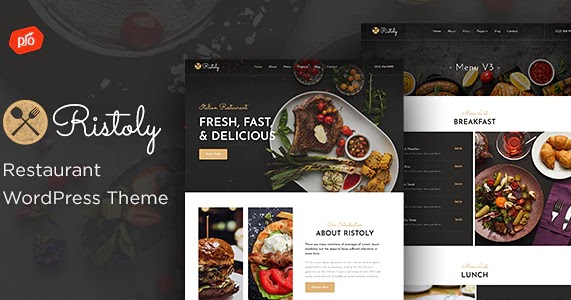In this image, the left side features a prominent white text that reads, "Boris Dolly Restaurant WordPress Theme," indicating that this is a specialized WordPress theme designed for restaurant websites. The blurred background highlights a food-related page, enhancing the theme's culinary focus. 

At the center of the image, a spotlight shines on a page displaying the slogan, "Fresh, Fast, and Delicious," accompanied by a mouth-watering photograph of a sizzling meat steak, garnished with red tomatoes and green vegetables on a pristine white plate. Beneath this, the text "About Boris Dolly" introduces a section with a compact black description and additional enticing images of a burger and other culinary delights.

In the background, another image peeks through on the left side, labeled "Menu V3." Despite being partially obscured by the foreground content, it reveals a detailed breakfast and lunch menu layout. The breakfast segment includes silverware icons—a fork and knife—alongside an arrangement of brown bread dough and two plates, one brown and one white. The lunch section is set against a white backdrop with black text. 

Noteworthy details include the restaurant's logo featuring a circle with a fork and spoon crossed in the center, and the top left corner prominently displays the label "PRO" in bold, white letters against a red background. Together, these elements present a comprehensive and visually appealing preview of the Boris Dolly Restaurant WordPress Theme.